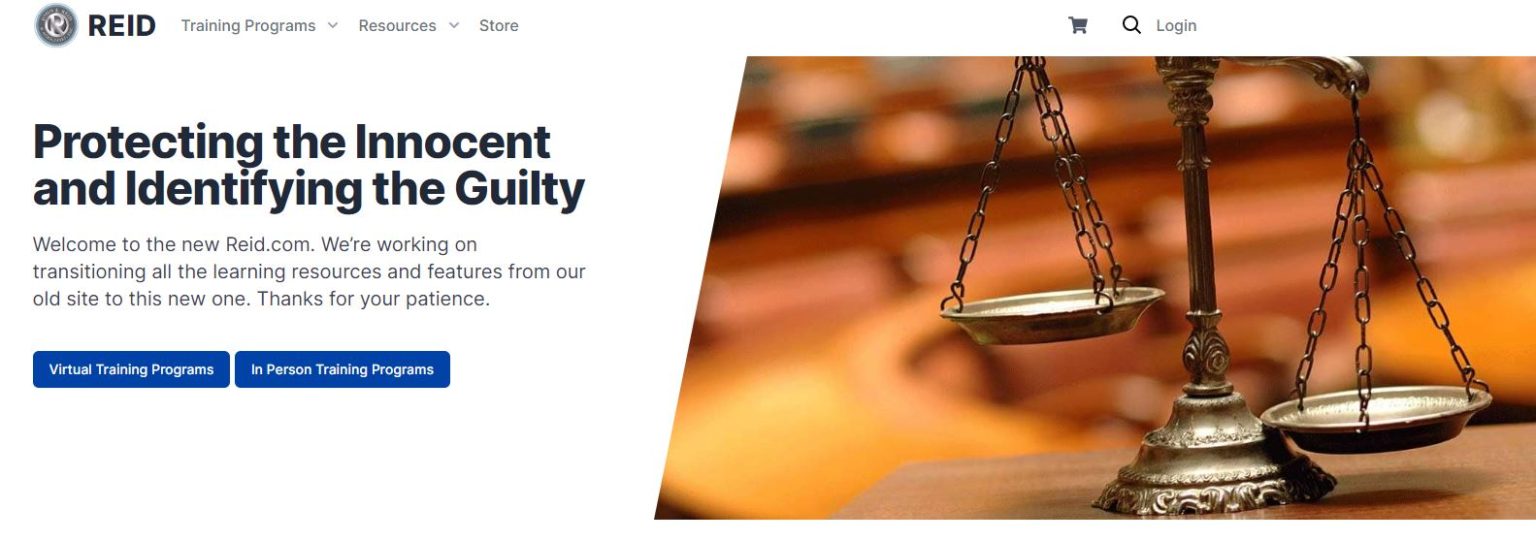This image is a cropped screenshot of the READ homepage, primarily focusing on the upper section. In the top left corner, the READ logo is prominently displayed. To its right, there are three main navigation categories: "Training Process," "Resources," and "Store." Further to the right are two icons: a shopping cart and a login icon. Below this navigation bar, there is an image with an angled design on the left side, slanting towards the right. Adjacent to the image, on the left, is a succinct description of the website in dark blue letters, accompanied by a small paragraph in smaller blue text. Two buttons are positioned beneath this text description; the button on the left reads "Virtual Training Program," while the button on the right says "In-Person Training Programs." The lower portion of the homepage is not visible in this cropped screenshot.